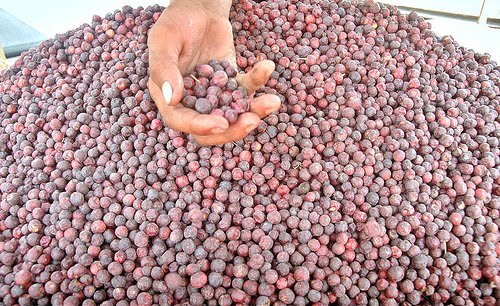The image depicts a large, vibrant pile of small berries, primarily characterized by a range of shades from light pink, through various hues of red, to dark purple. Among these berries, whose colors suggest they might be cranberries or a similar fruit, there's a prominent human hand grasping a handful of them. This hand, belonging to an African-American individual, is a striking focal point with upturned, curled fingers and white nail polish on the thumb, extending from the top center of the image and reaching into the mound. The photo is brightly lit, emphasizing the glossy, unwashed texture of the berries, and appears to be taken from an overhead perspective. Background details include a blue area in the upper left quadrant and a white area in the upper right quadrant, suggesting a glass or white surface on which the berries are spread. The overwhelmingly dominant feature of the image is the mounded berries, which occupy nearly the entire frame.